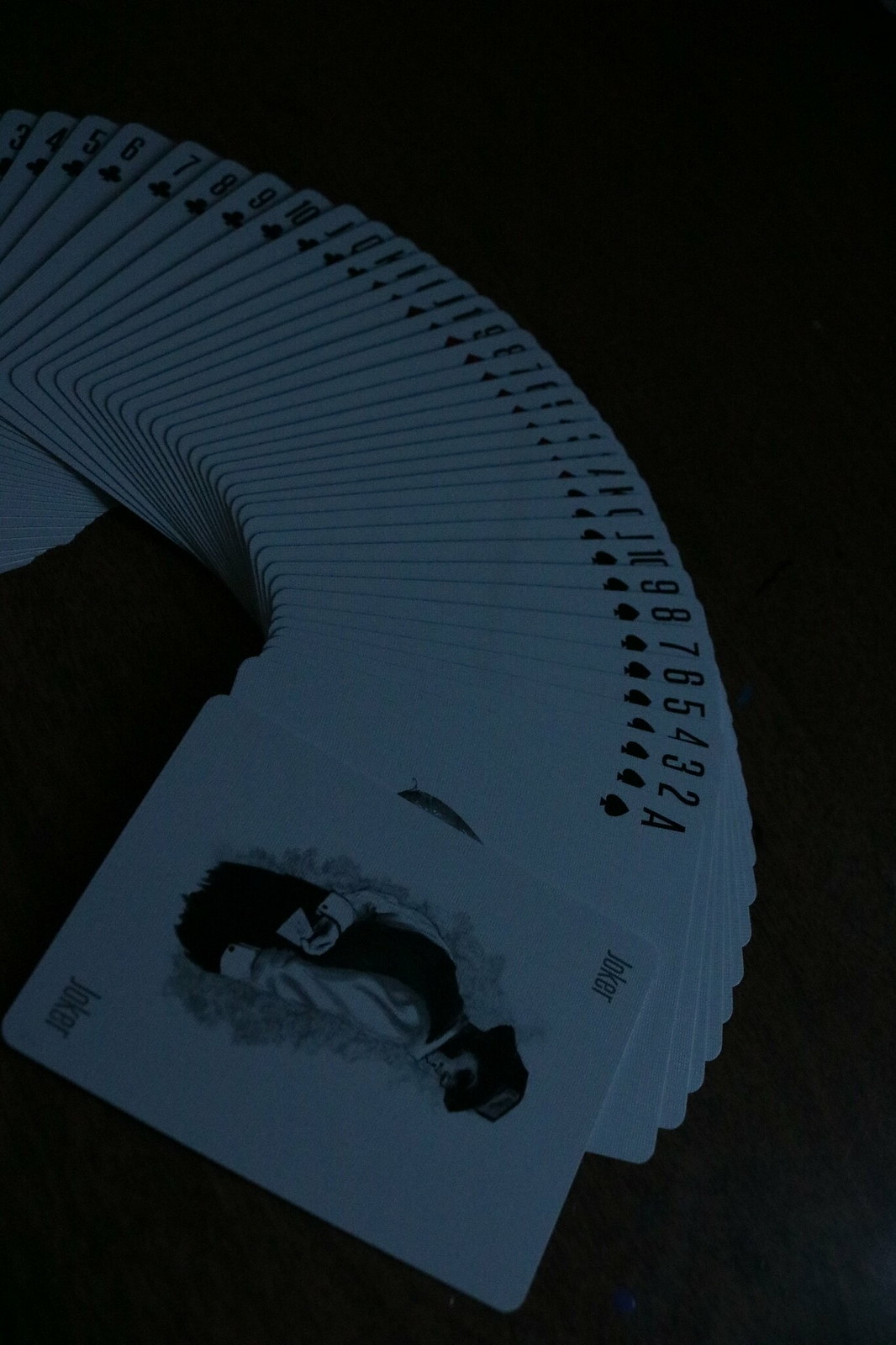The image features a mesmerizing spread of playing cards, elegantly arranged in a semicircle on a caramel-colored marble table. The cards are exclusively from the spades and clubs suits, all showcasing a pristine white color. The layout extends beyond the frame, suggesting an abundance of additional cards.

At the forefront, positioned prominently on the right side, is a card depicting a figure identified as the Joker. This card displays the image of a male figure adorned in a fancy white shirt, complemented by a black vest and a stylish black hat, almost inverted from the viewer’s perspective.

Starting from the Joker and extending upwards, the sequence of cards unfolds with the ace of spades, followed numerically by 2, 3, 4, 5, and so on. The middle section of the spread features indistinct cards, though their black coloration and spade-like pointed edges remain visible. Transitioning seamlessly into the clubs, the cards continue their numerical descent with the queen, jack, 10, 9, 8, 7, 6, 5, 4, and 3 in visible succession, curving downwards in the elegant arc. The combination of the detailed arrangements and the luxurious marble backdrop creates a captivating visual tableau.